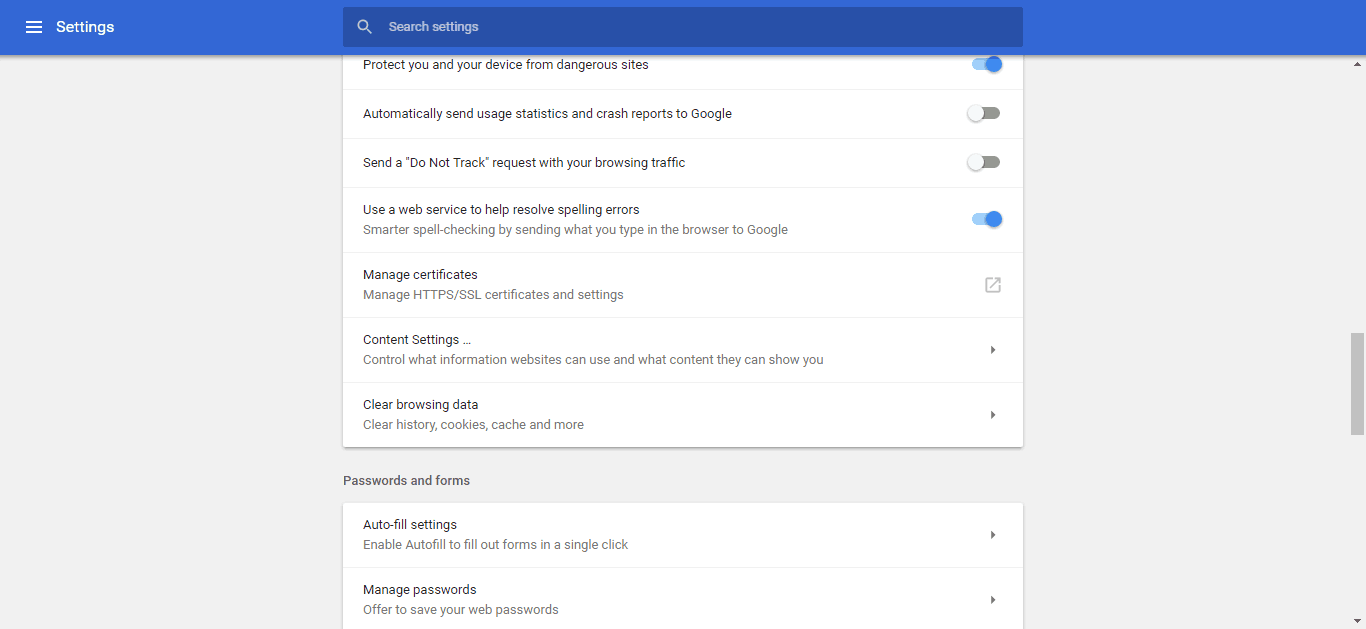Screen capture of a settings page within a browser. The top left corner clearly shows the word "Settings," and to its right is a prominently placed search bar labeled "Search settings." The partial scroll obscures the heading for the current section of settings being displayed. 

The visible settings options include:

1. **Protect you and your device from dangerous sites:** The toggle switch to the right is enabled.
2. **Automatically send usage statistics and crash reports to Google:** The toggle switch to the right is disabled.
3. **Send a "Do Not Track" request with your browsing traffic:** This setting is also turned off, with the toggle switch to the left.
4. **Use a web service to help resolve spelling errors:** The associated toggle switch is enabled.

Following these settings, there are additional options listed without toggle switches:

- **Manage certificates**
- **Content settings**
- **Clear browser data**
- **Passwords and forms**

At the bottom, a new section starts with:

- **Autofill settings**
- **Manage passwords**

This settings page appears to be from a web browser, possibly Google Chrome, given the mention of Google-specific options. It offers various controls to enhance security, privacy, and user experience by customizing the behavior of the browser.